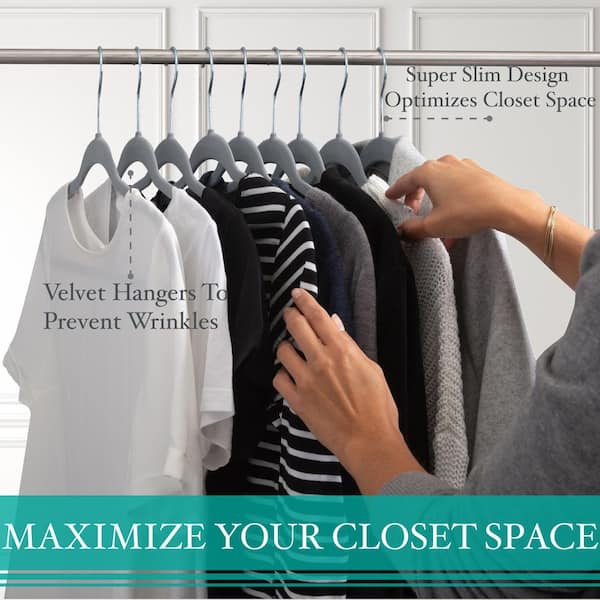The image features an advertisement showcasing velvet hangers with a super slim design, aiming to optimize closet space. A fair-skinned woman, wearing a gray outfit and a gold bracelet, is seen sorting through clothes on the hangers. The gray, black, white, and black-and-white-striped garments hang neatly on a metal rod against a white wall. Key phrases like "Super Slim Design Optimizes Closet Space" and "Velvet Hangers to Prevent Wrinkles" are prominently displayed, with "Maximize Your Closet Space" highlighted in white lettering on a green background at the bottom of the image, reinforcing the product's space-saving benefits.